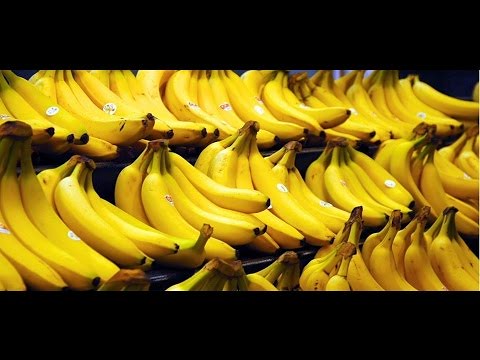The image depicts a collection of numerous bright yellow banana bunches, organized in three distinct, tiered rows against a black background. Each row features approximately 5 to 8 bunches, with each bunch containing around 5 to 7 bananas. The bananas are primarily ripe with golden yellow skin, some displaying small brown specks or bruises, particularly on the edges and stems where they conjoin into a brown spot. Each banana is marked with a white sticker featuring text or a picture, further enhancing their detail. The arrangement appears deliberate, with the bananas stacked in a stair-like fashion, creating a visually appealing, orderly display of the fruit.